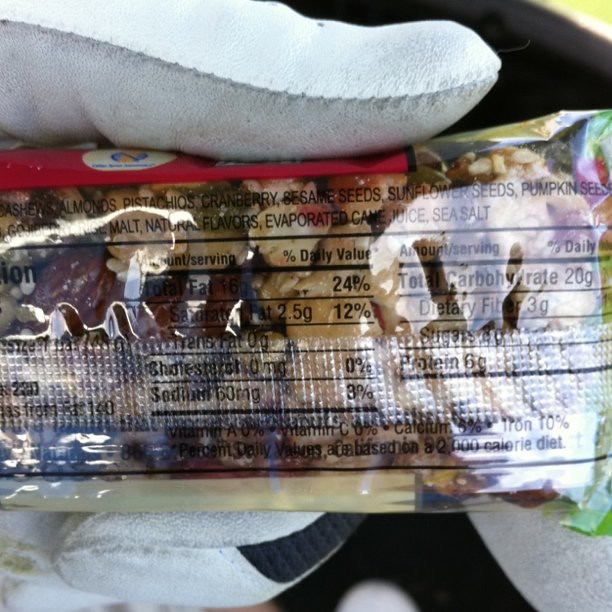A detailed first-person perspective image captures the back of a clear muesli bar packet, allowing visibility of the nut-filled muesli bar inside. The picture is taken with the right hand, while the left hand, clad in a glove with grey finger pads and a white top, holds the packet. The back of the packet prominently displays a nutritional table. Key nutritional information includes: total fat at 16 grams (24% daily value), saturated fat at 2.5 grams (12% daily value), trans fat at 0 grams, cholesterol at 0 milligrams (0% daily value), sodium at 60 milligrams (3% daily value), and total carbohydrates at 20 grams. Additionally, the bar provides 3 grams of dietary fiber, 8 grams of sugars, and 6 grams of protein. Other vitamins and minerals listed are vitamin A at 0%, vitamin C at 0%, calcium at 6%, and iron at 10%. The daily percentage values are indicated as being based on a 2,000-calorie diet, although some daily value percentages are cut off due to the design of the packet extending beyond the visible area.